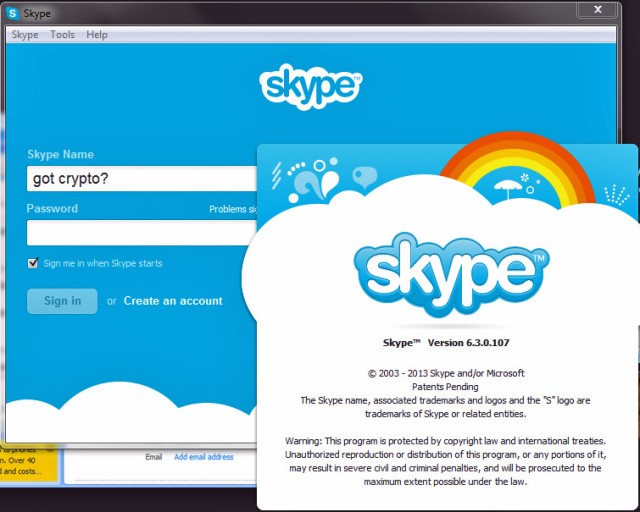The image is a screenshot of Skype's homepage. At the top, there is a horizontal black border. On the left side of this border, there is a blue square featuring a white 'S'. Next to this square, the word "Skype" is written in black with a slightly hazy gray outline. Towards the right end of the black border, there is a white 'X'. A vertical black border runs down the right side of the image for about three inches, next to which there is a pop-up tab.

Below this, at the top of the page, there is a gray border. On the left side of this border, the word "Skype" is written in black, followed by the options "Tools" and "Help". The main background of the page is a gradient blue sky with a few clouds visible two inches from the bottom. In the center, the word "Skype" appears in light blue, enclosed within a thick white border.

Further down, to the left, the word "Skype" appears again in white. Adjacent to this, inside a black rectangle, the partially cut-off text reads "Got crypto?" This area features another pop-up tab continuing down to the bottom of the screen and stretching across the page. To the right, "Password" is written next to a rectangular input field. Below this, there is a gray square with a black checkmark and the text "Sign me in when Skype starts."

Near the bottom, there is a dark blue tab with the options "Sign in" and "Create account" visible in a lighter blue. Another pop-up appears lower down, featuring a rainbow with a bit of sky above it and a white cloud occupying the bottom two-thirds. This section has a white background, a blue border around "Skype," and additional information about the platform, including its version, dates, and patents pending details, along with the Skype name and logo.